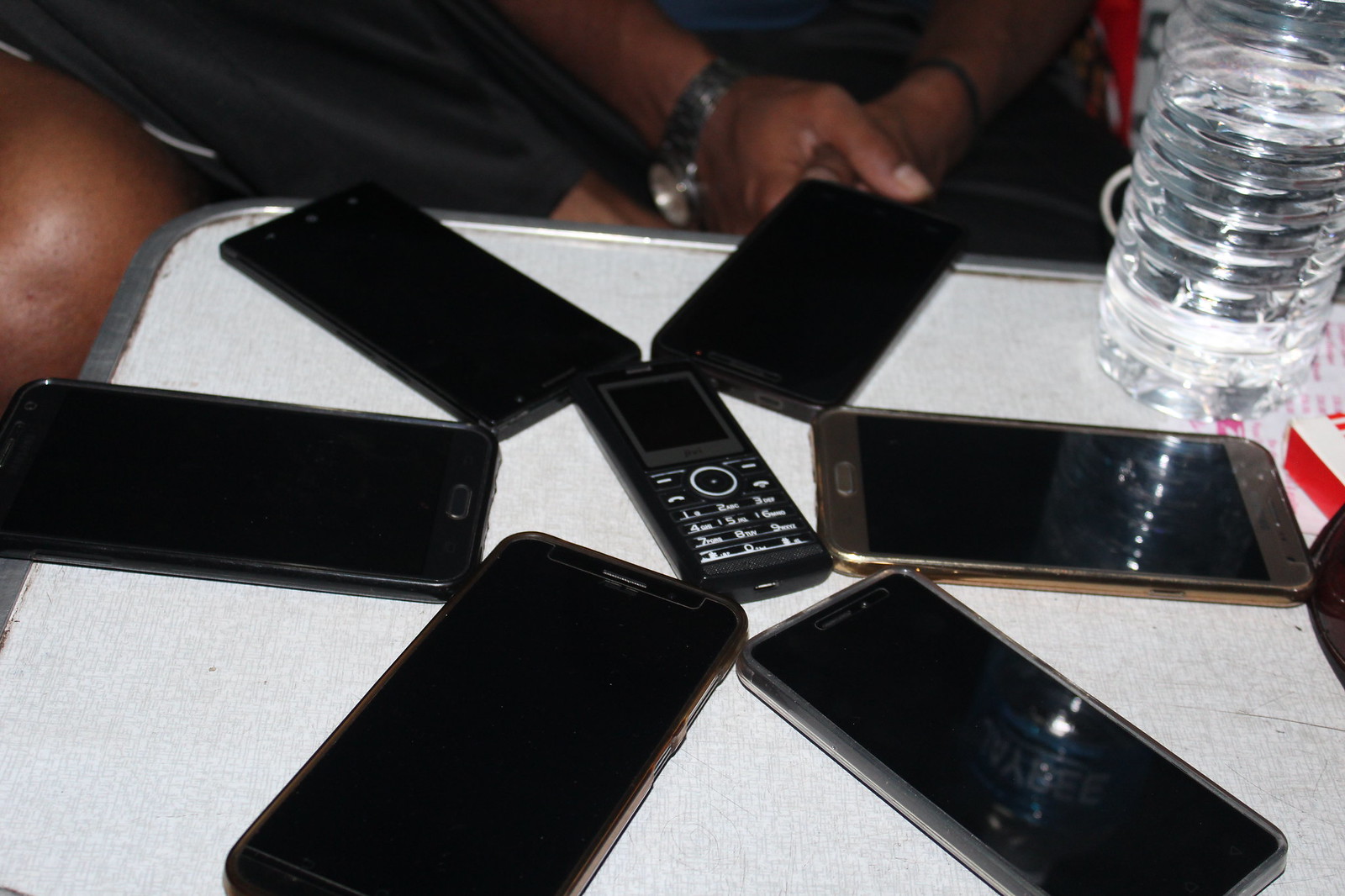The photograph displays an overhead view of a white, square table featuring a hexagonal arrangement of six smartphones with an older non-smartphone at the center. The older phone, characterized by its traditional key face and small top screen, is the focal point, surrounded symmetrically by the six smartphones with black screens. The table has a metallic rim, and there is a partially filled plastic water bottle positioned at the top right corner. At the very top of the image, an African-American man is partially visible, showing only his arms and leg. He wears a watch and appears to be holding the smartphone that is at the uppermost position in the arrangement. The whole setup creates a star-like or flower-petal pattern of modern devices encircling the central, more dated phone.